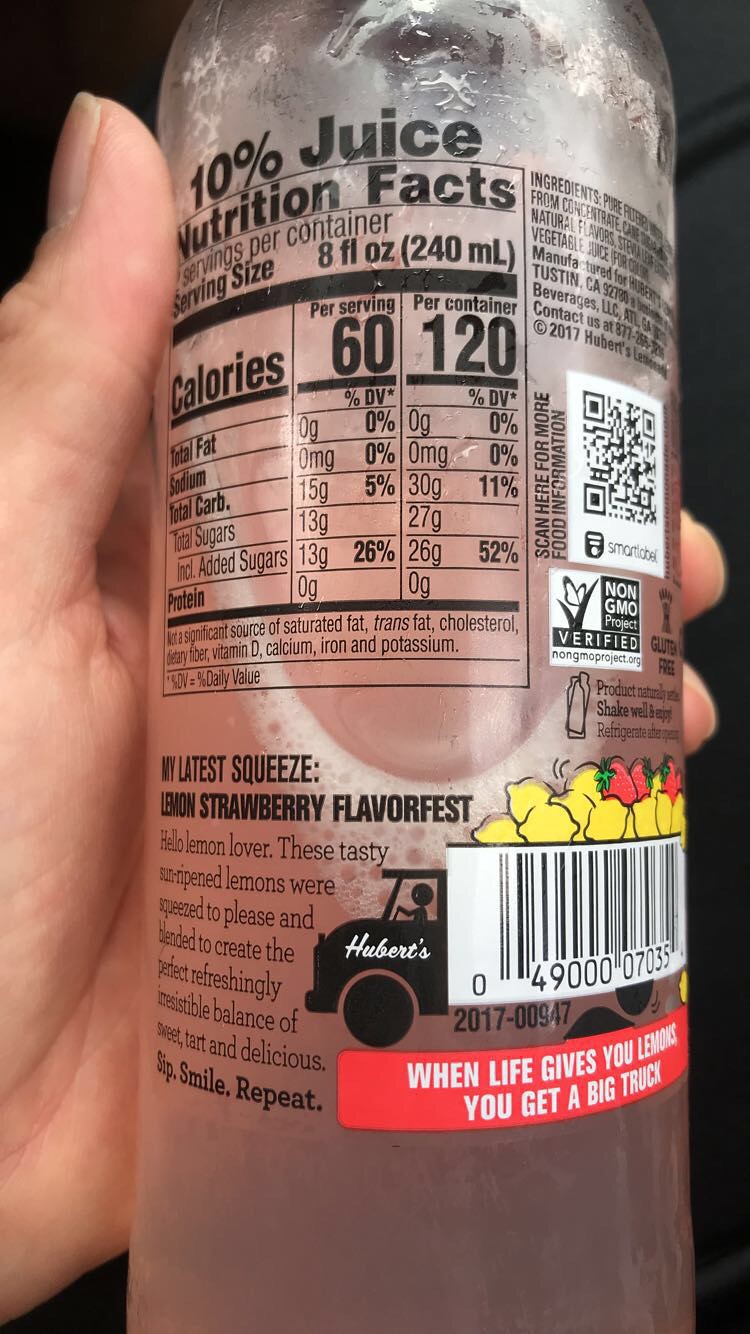A close-up image captures a hand holding a bottle of flavored water, specifically lemon strawberry flavored, by its box-like packaging. The bottle is gripped in the left hand, with the thumb visible on the side and the tips of the pointer and middle fingers peeking out from behind. The focus is on the back of the box, prominently displaying its nutrition facts:

- **Serving Size**: 8 fl oz (240 ml)
- **Servings Per Container**: 2
- **Calories**: 60 per serving (120 per container)
- **Total Fat**: 0g
- **Sodium**: 0mg
- **Total Carbohydrates**: 5% per serving, 11% per container
- **Total Sugars**: 25% added sugar per serving (26g total, 52% per container)
- **Protein**: 0g

Additional details note that the product is not a significant source of saturated fat, trans fat, cholesterol, dietary fiber, vitamin D, calcium, iron, or potassium.

Beneath this, a playful marketing tagline reads, "My Latest Squeeze: Lemon Strawberry Flavor Fest. Hello Lemon Lover. These tasty sun-ripened lemons were squeezed to please and blended to create the perfect, refreshingly irresistible balance of sweet, tart, and delicious. Sip, Smile, Repeat."

To the right, near the barcode, a whimsical graphic turns the barcode into the back of a truck. An illustrated driver is seen at the front, with the brand "Hubert's" above and the phrase "When life gives you lemons, you get a big truck" below. A QR code also sits on the left-hand side of the bottle.